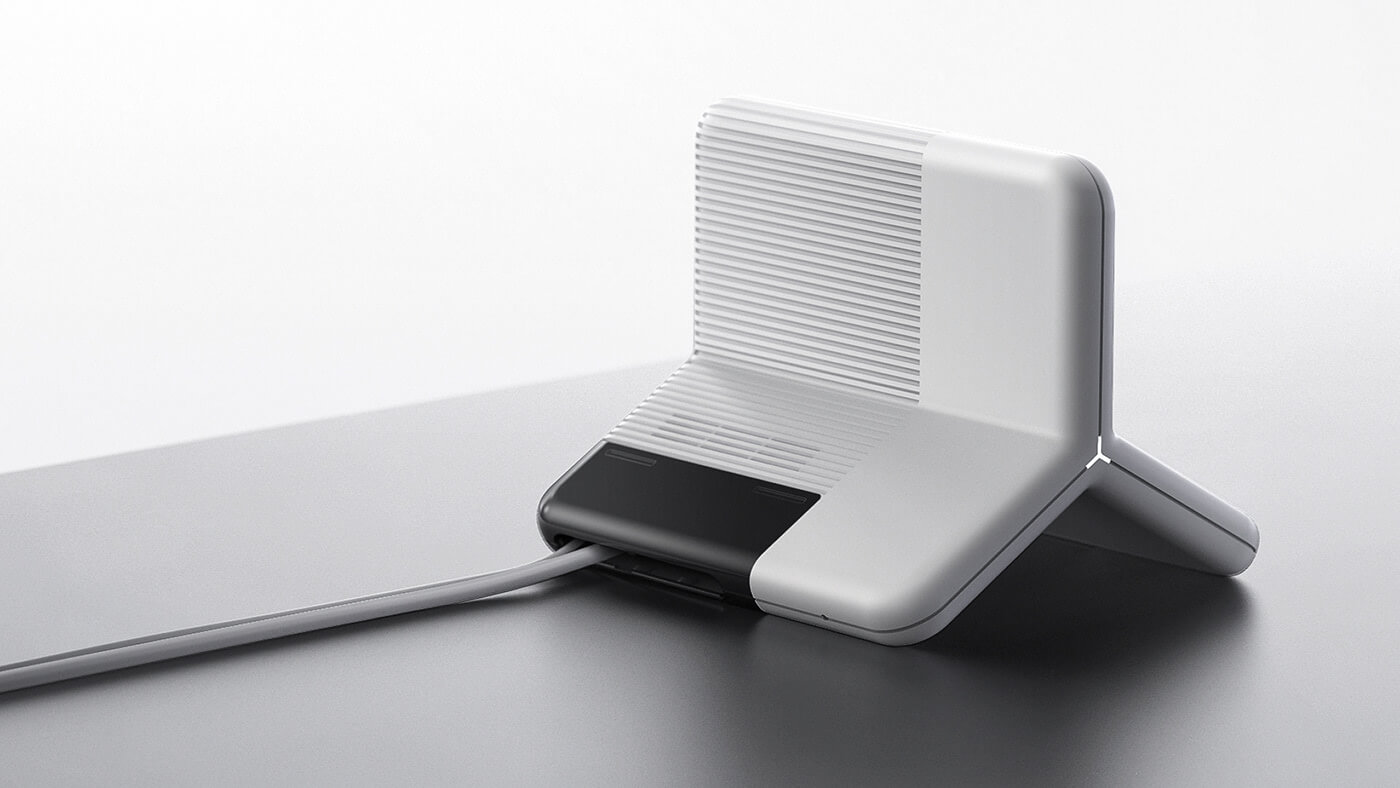The image captures a white, plastic electronic device resting on a metallic-looking, gray table, which subtly directs the viewer's gaze towards the device through its reflective highlights. The device itself, appearing clean and sleek, has a distinctive shape resembling a Y or a jack with three equal-length extensions sprawled out to its sides. This unique "Y" shape features airflow vents or slats along its sides, hinting at a function related to cooling or ventilation. The device sits more towards the right in the photo, casting a shadow downward, and from its bottom extends a black rectangle with a cord emerging from it, trailing horizontally to the left and out of the image. The background contrasts subtly with a gradient from gray to white, enhancing the visibility of the device's details under the overhead light source.